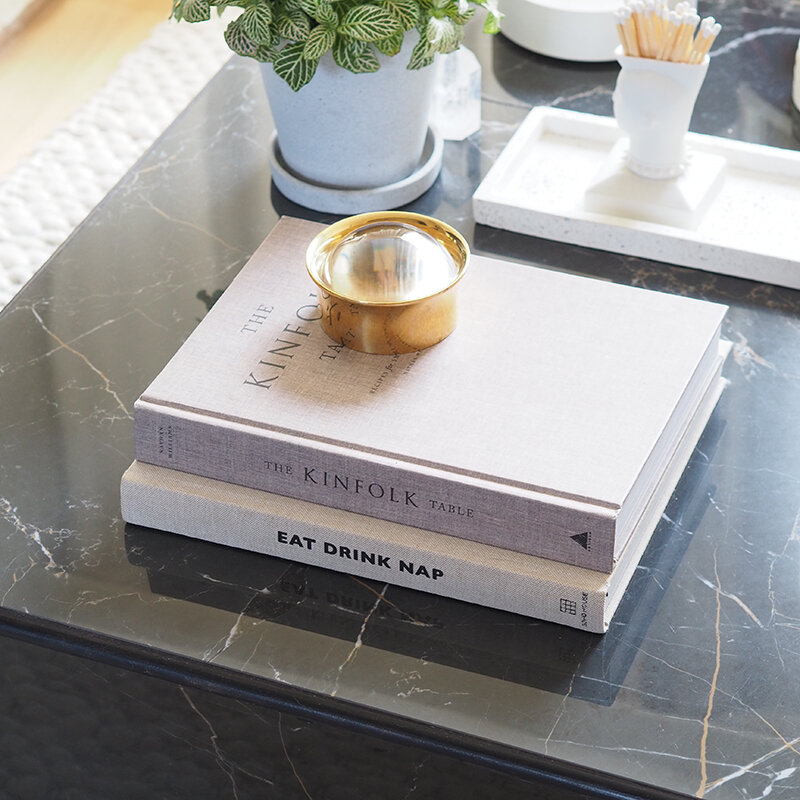This indoor color photograph showcases a sleek, dark marble countertop intricately veined with white lines. Central to the composition, two hardcover books with white covers are neatly stacked. The top book, titled "The Kinfolk Table," is topped with an intriguing golden, reflective cup that appears to hold a bubble. Below it, the book titled "Eat, Drink, Nap" can be seen. To the upper left of the books sits a white pot containing a lush green plant with delicately veined leaves, complemented by a matchingly white tray designed to collect water. To the right of the plant, a long rectangular white tray holds a small container filled with tan-colored Q-tips. In the background, partially out of view, are a white bowl and a glass bottle. The photograph also captures a glimpse of light wood flooring in the top left corner, adding warmth to the otherwise cool-toned setting.